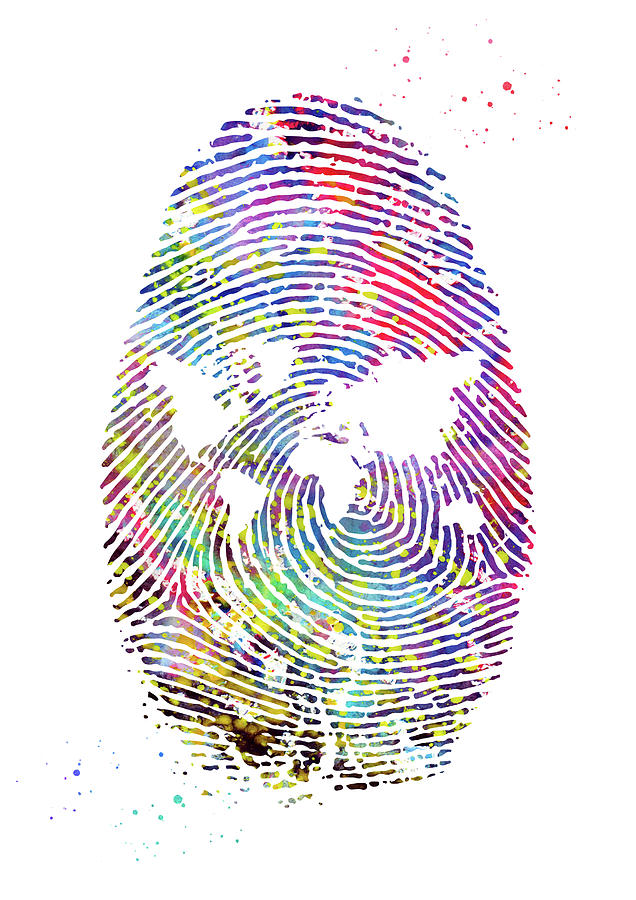This artwork features a vibrant and intricate fingerprint, its lines painted in a riot of colors including shades of red, green, purple, teal, yellow, blue, and darker hues. The fingerprint is set against a white background, with seemingly random yet artfully splattered colors extending to the upper right and lower left corners, predominantly in red, green, and blue. What sets this print apart is the clever integration of the seven continents outlined within the fingerprint’s core, carved out in pristine white space. Detailed shapes of the Americas, Europe, Africa, and other continents stand out vividly amidst the colorful swirls, symbolically connecting the uniqueness of one's identity to the vastness of the world, suggesting a message about the global nature of individuality.